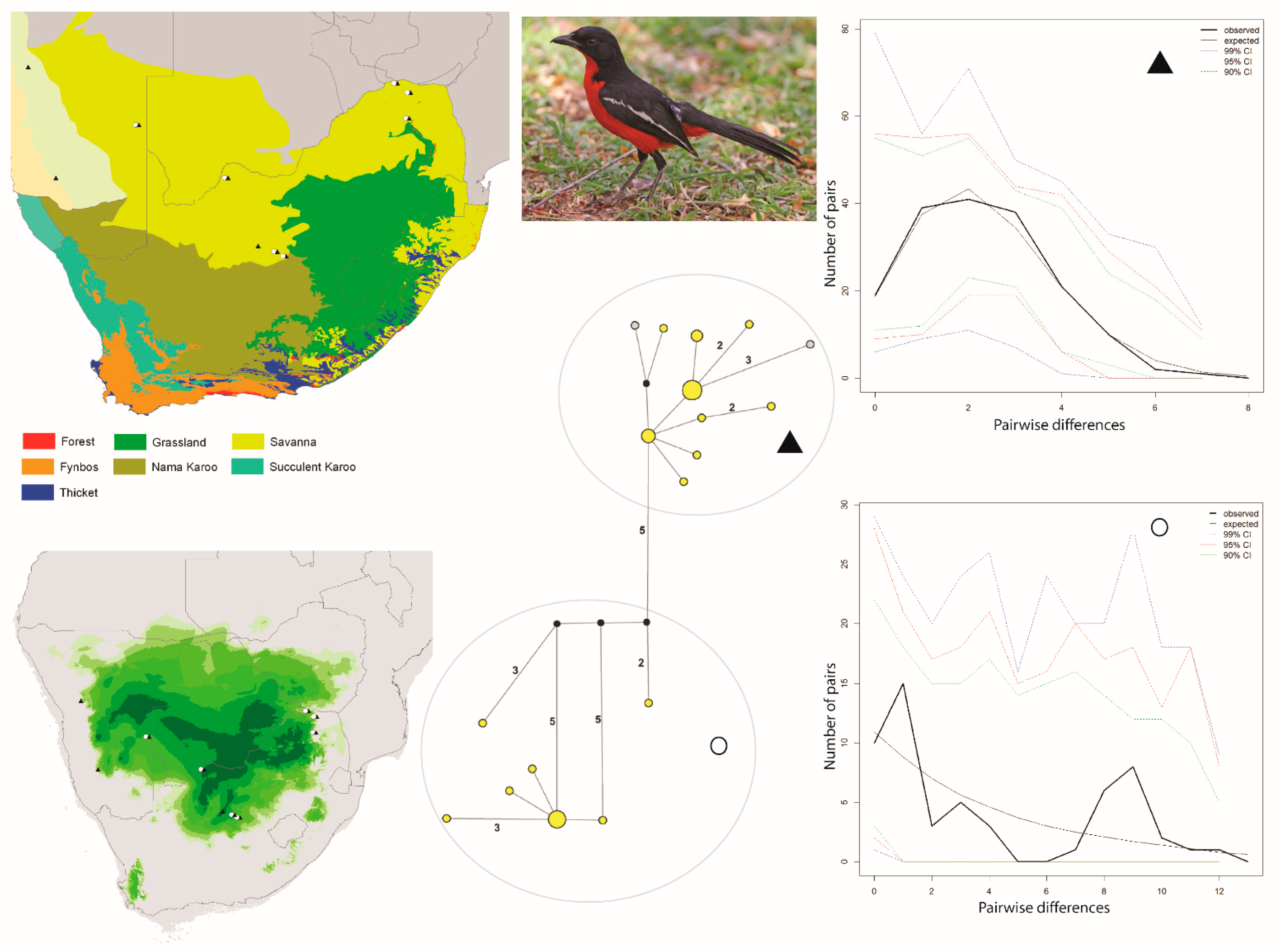The image features a series of scientific diagrams and visuals. In the top left corner, there is a detailed map of South Africa, color-coded with a legend beneath it. The map designates various ecological zones: yellow for savannah in the upper regions, green for grassland on the right, red for forest scattered in the bottom right, orange for finboss in the bottom left, olive green labeled nama karu in the central bottom left, teal aqua green for succulent karu along the left-hand coast, and dark blue marking thicket areas also in the bottom right. To the right of this map, there is a vivid photograph of a bird on a grassy surface, characterized by its red belly, black back, a white stripe on its wings, black eyes, a black beak, and a long black tail.

To the right of the bird photograph, there are two graphs, both featuring lines with a downward slope from the top left to the bottom right. These are enclosed in a black frame, with the y-axis labeled 'Number of Pairs' and ranging in the first graph from 0 to 80 and in the second, smaller scale graph from 0 to 30. The x-axis on both graphs is labeled 'Pairwise Differences', ranging from 0 to 8 on the first graph and from 0 to 12 on the second.

Beneath the graphs, in the bottom right corner, is another map of South Africa, depicted in varying shades of green, indicating different measures, possibly of vegetation density or precipitation levels. To the left of these graphs, there is a complex diagram showing two circles stacked vertically with yellow circles branching out from them, connected by brown lines and marked with various numbers such as 2, 3, 5. Alongside this, there are a black triangle and another black circle with a white interior, suggesting some form of hierarchical or relational structure.